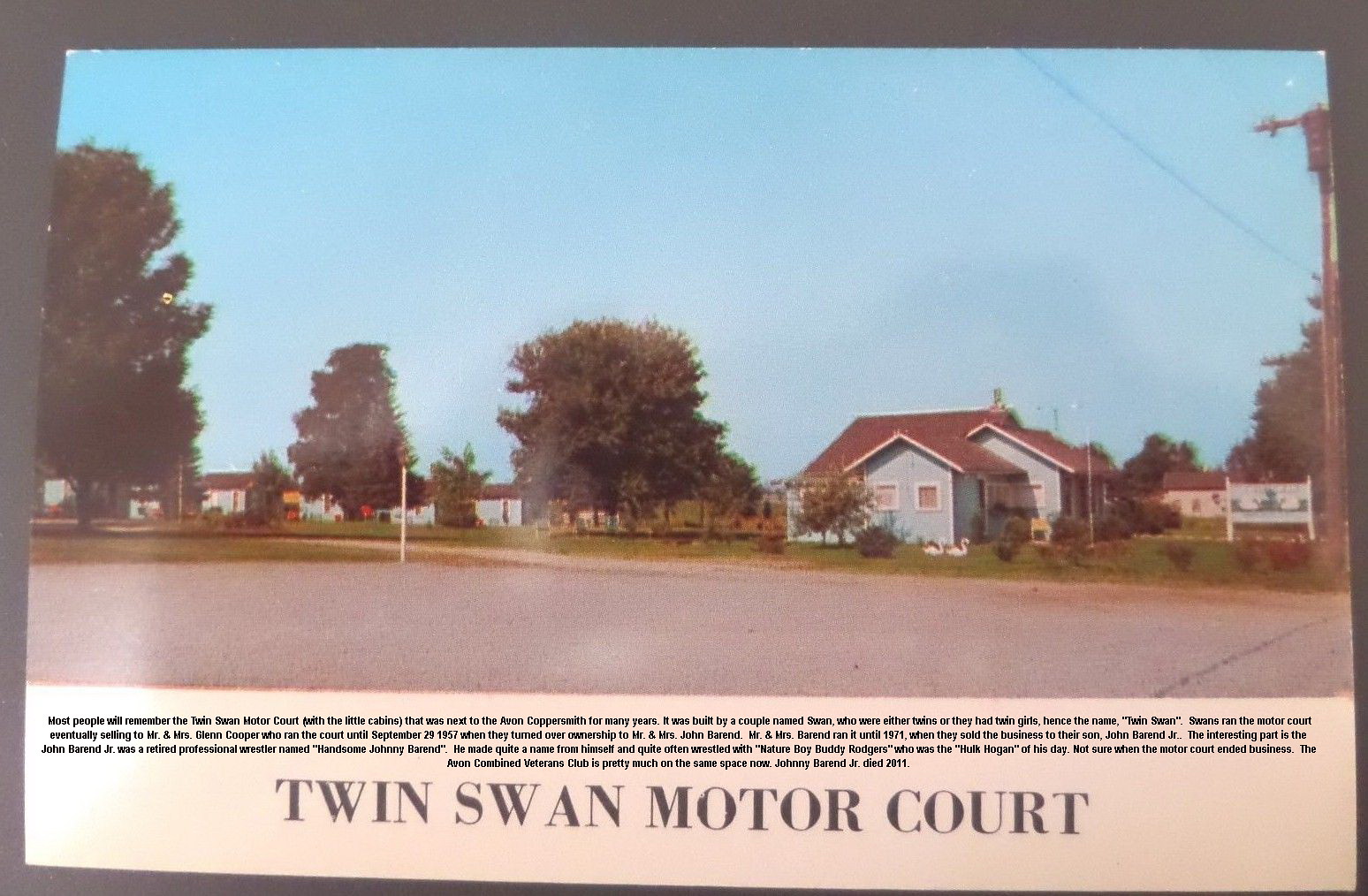The image appears to be an aged advertisement for Twin Swan Motor Court featuring a serene neighborhood scene. Dominating the right-hand side is a pale blue house with a brown roof and a well-maintained lawn in front. Outside the house, two swans or flamingos can be seen, adding to the tranquil setting. The sky is a clear, pure blue, indicative of a pleasant summer day. To the left of the house are several trees, including one notably large tree, which contribute to the picturesque quality of the neighborhood. Behind the trees, smaller cabins are visible, suggesting additional accommodations. In front of the house runs a sidewalk and a concrete road. The bottom section of the image features a white rectangular box with small, difficult-to-read black print and is bordered by a larger black frame. Prominently displayed in bold, silver-colored, capital letters beneath the photo is the text "TWIN SWAN MOTOR COURT," signifying the name of the advertised location.